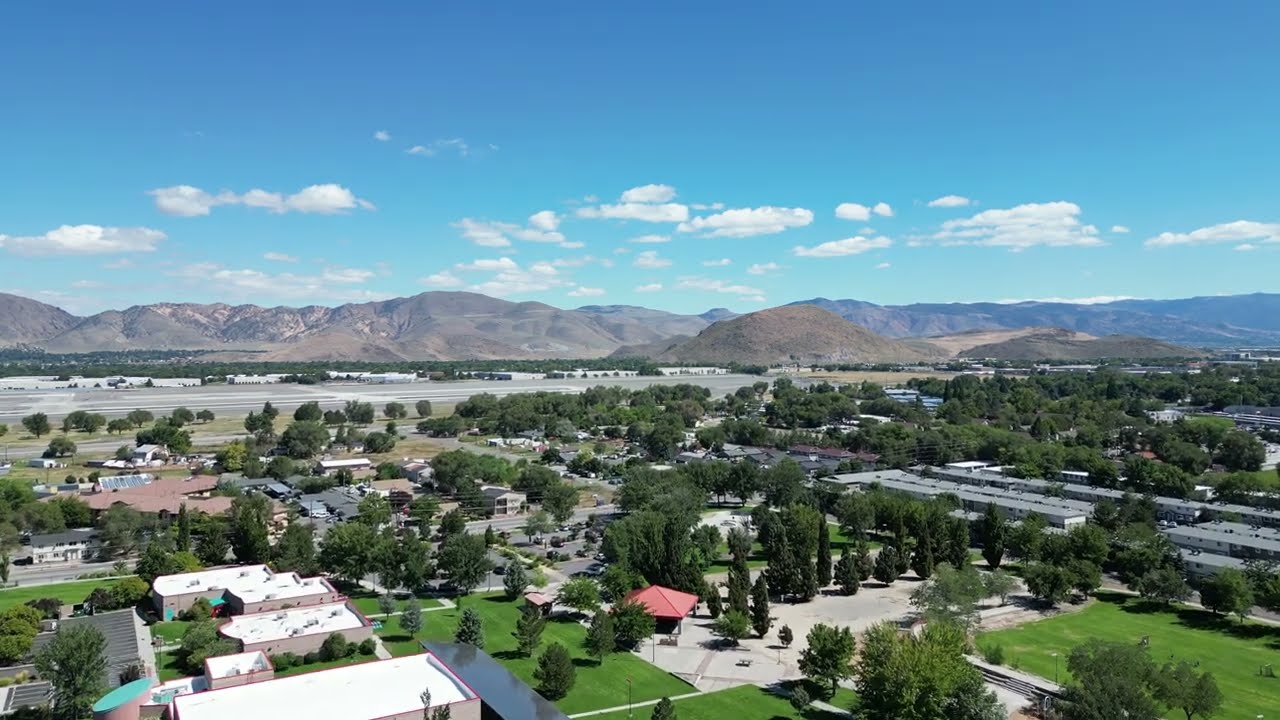This photograph, taken from an elevated vantage point, offers a sweeping view of a town characterized by predominantly white, flat-roofed houses interspersed with well-kept green gardens and abundant trees. The neatly manicured grass and verdant, towering trees add to the town’s lush appearance, which creates a striking contrast against the various residential and square-shaped buildings scattered throughout. Towards the lower left, a larger square building, possibly a manufacturing or non-residential structure, stands out among the homes. In the distance, the brown hills form a natural backdrop, and above them, the expansive blue sky is dotted with a few clouds, providing a picturesque horizon line. The overall impression is of a tranquil, green town nestled at the base of scenic hills, viewed from a high perspective that could be achieved with a drone.